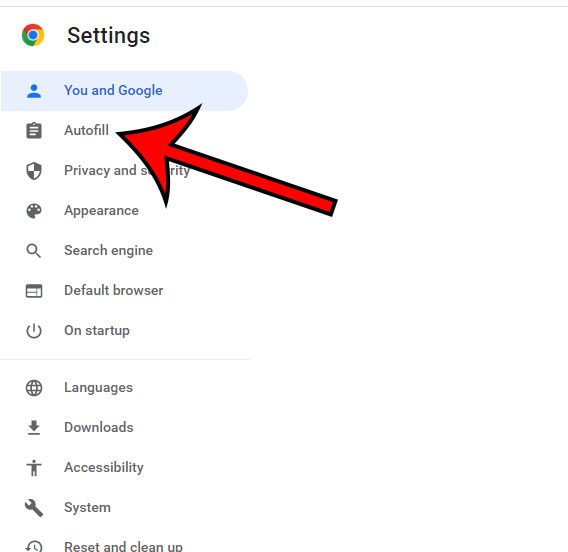The image displays a Google settings page with a predominantly white background. On the left side, a single column features the Google icon and the word "Settings" at the top. Below this heading, several menu items are listed. The first item, "You and Google," is highlighted with a light blue and blue font color. The subsequent items—"Autofill" (which is marked by a large red arrow pointing towards it), "Privacy and Security," "Appearance," "Search Engine," "Default Browser," and "On Startup"—appear in gray text against the white background. Following "On Startup," a thin gray line separates the next set of options: "Languages," "Downloads," "Accessibility," "System," and "Reset and Cleanup," each with corresponding icons. A light gray horizontal line spans the top of the image for additional separation. There are no other visible marks on the image.